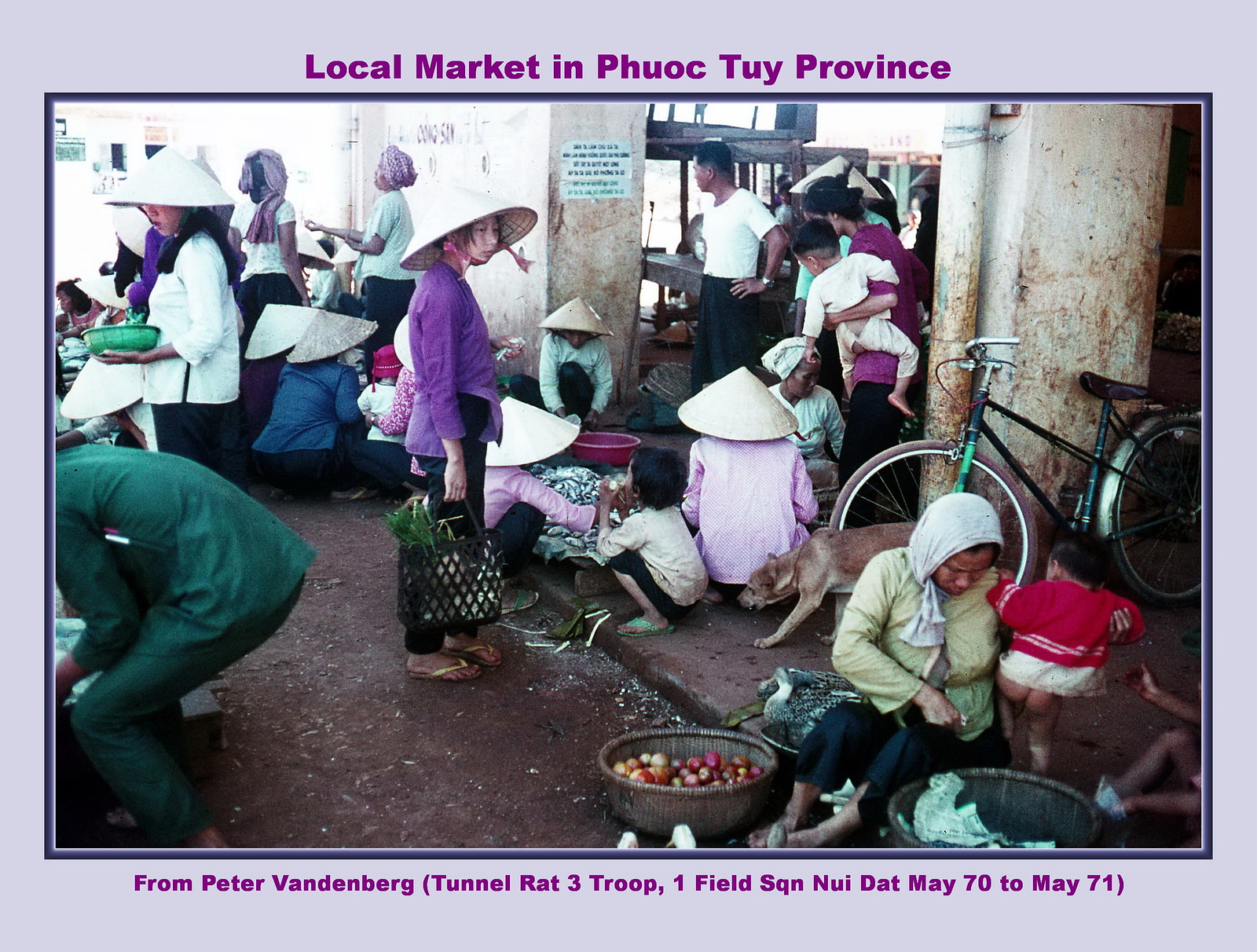The photograph captures a bustling local market in Phuoc Tuy province, framed by a soft pastel pink or violet border with bold purple text at the top reading "Local Market in Phuoc Tuy Province." The bottom text, also in purple, states, "From Peter Vandenberg, Tunnel Rat 3 Troop, 1 Field Squadron, Nui Dat, May 70 to May 71." The scene is filled with vibrant activity, primarily involving women and children, with a few men scattered throughout. Most people are wearing traditional conical rice hats. The market is dense with baskets of fruit, vegetables, and produce, some children and people selling fish. In the center right, a bicycle leans against a wall, while a young girl, dressed in a purple top, black pants, and yellow flip-flops, stands carrying a black netted basket. In the foreground, a woman in a yellow top and headscarf sits on the curb with a half-naked child, and a dog nearby sniffs around, possibly for food. The image encapsulates the daily life and communal hustle of an Asian marketplace.